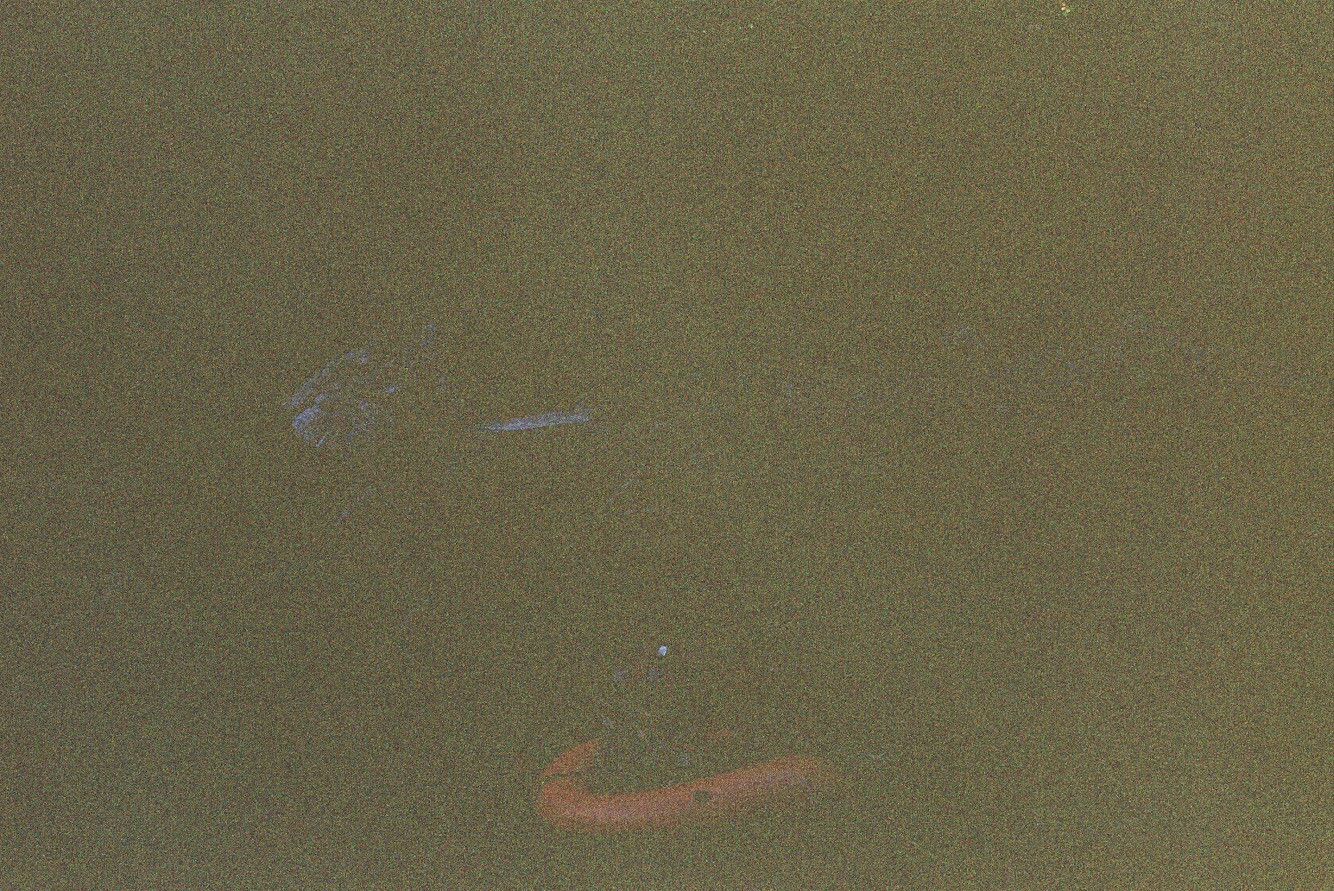The image features a predominantly grainy, brown background with black undertones that creates a simple yet abstract scene. Scattered across this surface are hundreds of small, light dots and faint traces of white, blue, and a hint of yellow at the top, adding subtle layers of complexity. Near the center, there are light purple markings, while in the lower half of the image, a distinct reddish-orange, J-shaped figure emerges, reminiscent of a worm or a splash of paint. This obscure object seems to be either obscured or partially embedded within the textured background, which evokes different interpretations, such as a path in a park or a rubbery surface. The overall impression is one of minimalism, dominated by a rich, detailed brown canvas punctuated with sparse, colorful elements.